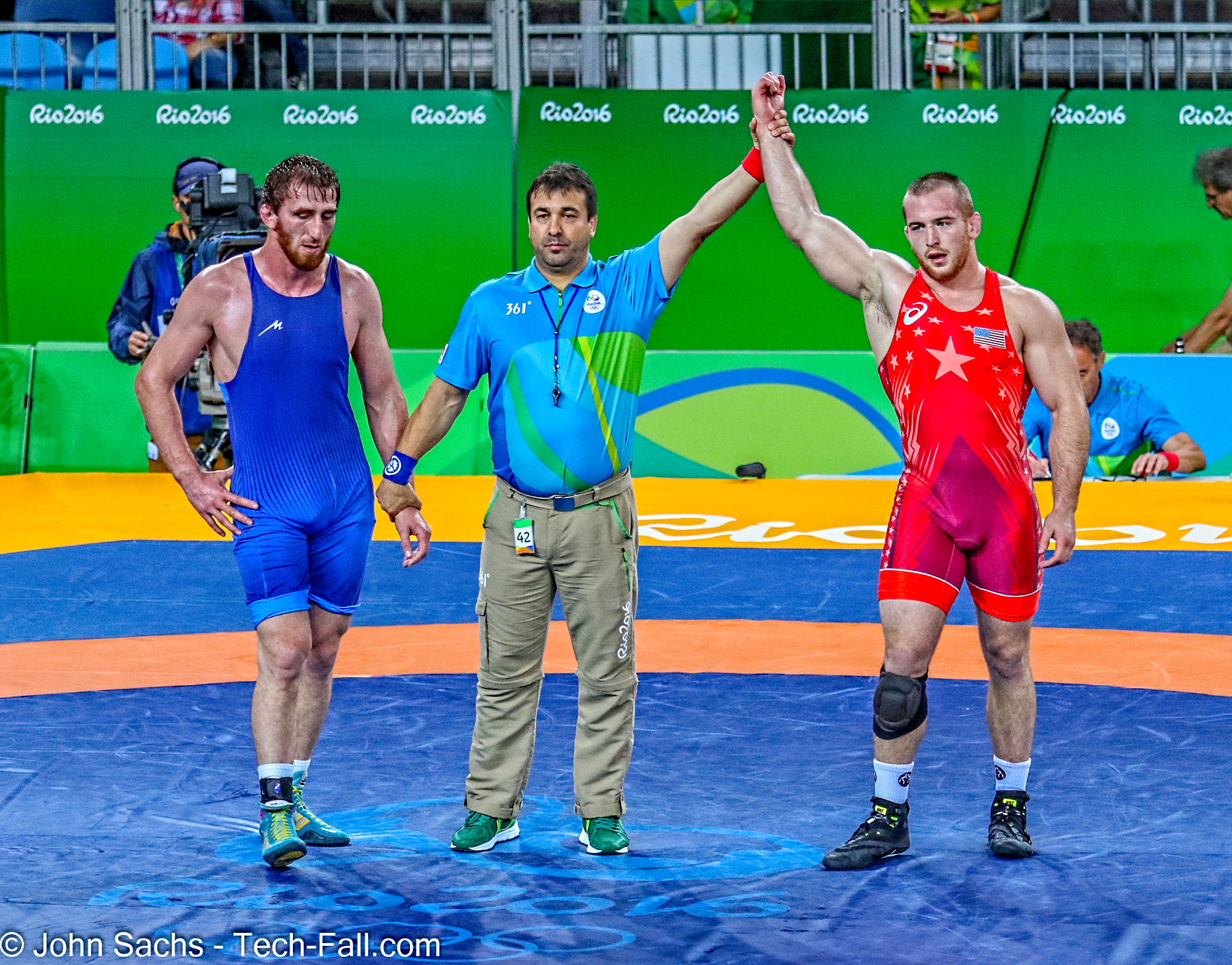In this vibrant photograph captured at the Rio 2016 Olympics, three men stand on a flat padded wrestling mat in the center of a gymnasium. The focal point is the referee, dressed in a blue shirt with green patterns and khaki pants, who is declaring the winner by raising the right arm of the wrestler on the right. This victorious wrestler sports a red uniform featuring a pink star in the center, a knee pad on his right knee, and a patch resembling the American flag on his left chest. His short buzz cut is noticeable against his triumphant expression. On the left, the defeated wrestler wears a blue uniform. The background reveals a bright green wall adorned with "Rio 2016" repeatedly, indicating the event's Olympic significance. Additional details include a man filming with a camera and another individual seated in a blue shirt. The bottom left corner of the image is marked with the text "John Sachs tech fail dot com."